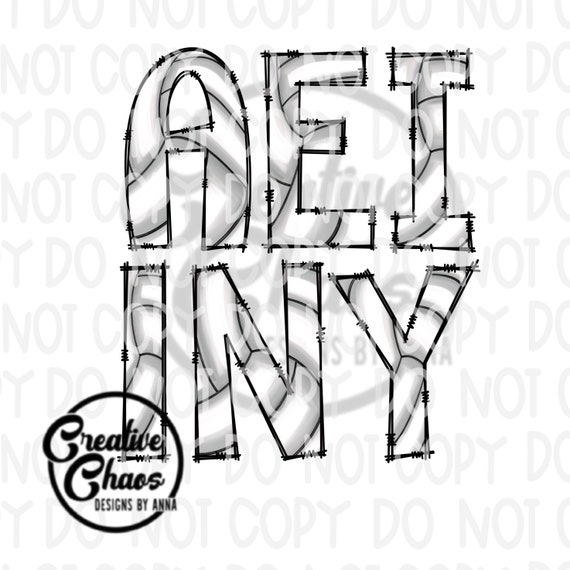This black and white, hand-drawn logo design features prominently the letters "AEI" on the top line and "INY" on the bottom line. The letters are intricately detailed, resembling barbed wire or patchwork, which adds a unique, textured effect. A graying, obtrusive watermark reading "do not copy" repeatedly overlays the entire design, making it challenging to discern finer details. In the bottom left, a circular logo reads "Creative Chaos Designs by Anna," with the same logo subtly echoed as a grayed-out watermark across the design. This artistic creation by Anna showcases a distinctive and somewhat cartoonish style with various shadings of gray and black lines. Despite the poor decision in watermark placement, the graphic boldly represents Anna’s creative endeavor.